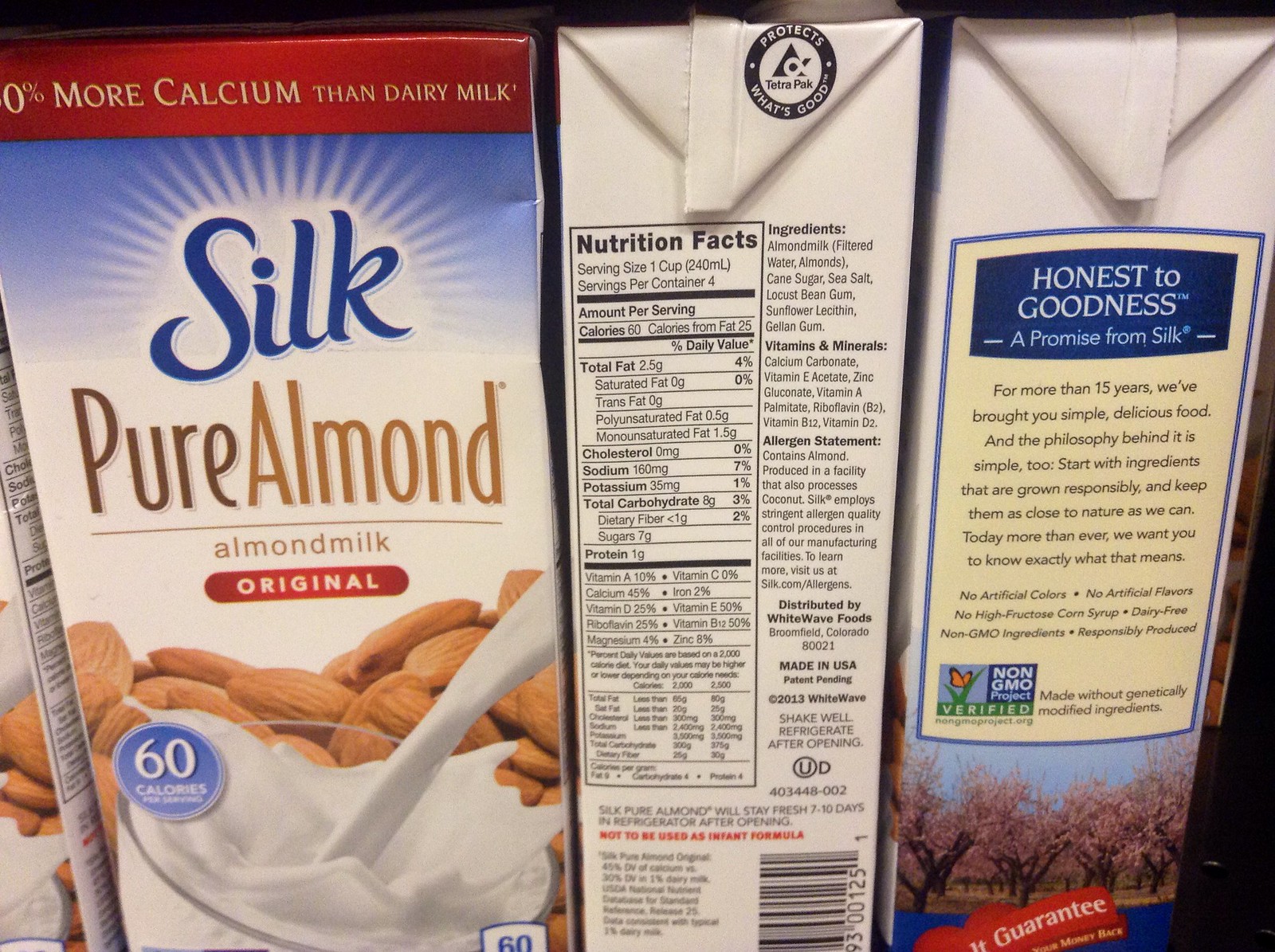This image is a detailed photograph of multiple boxes of Silk Pure Almond Almond Milk arranged on a shelf, showcasing the product from different angles. On the left, the front of a box of Silk Pure Almond Milk Original is prominently displayed. The carton features a red band at the top with text specifying its higher calcium content compared to dairy milk. Below, the iconic Silk logo is presented in blue, with "Pure Almond Almond Milk" in brown text underneath. Within a red oval, "Original" is clearly written in white lettering. The bottom of the carton depicts raw almonds and a splash of milk, emphasizing its almond-based origin, alongside a blue circle stating it contains 60 calories per serving.

The middle section of the photograph focuses on the side panel of the box where the nutrition facts are provided. Here, it details that one serving size is one cup, and there are four servings per container. The panel lists 60 calories per serving, with 25 calories from fat, along with other ingredients, vitamins, minerals, and an allergen statement ensuring comprehensive nutritional transparency.

On the right side of the image, another side panel is visible, featuring a blue box with white text that reads "Honest to Goodness, A Promise from Silk." This blue box is nested within a larger yellow rectangle that elaborates on the history of the product and highlights its non-GMO status. The careful arrangement of these boxes on the shelf not only showcases the front design but also gives viewers a comprehensive look at key nutritional information and branding promises.